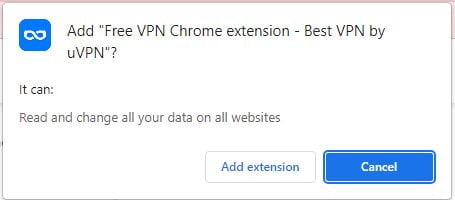This screenshot captures a section of the Google Chrome browser interface, specifically the prompt for adding a browser extension. The rectangular screenshot prominently features a medium blue icon in the top left corner, displaying a white infinity symbol (a sideways figure 8).

The main text reads: 'Add "Free VPN Chrome Extension - Best VPN by uVPN"?' which is surrounded by double quotation marks and punctuated with a question mark. Below this, a line of text outlines the extension's capabilities: 'It can: read and change all your data on all websites.'

At the bottom right of the screenshot, there are two clickable rectangular buttons with slightly rounded corners. The first button, in white with a light grey border, has blue text that reads 'Add extension.' The second button, colored blue with white text, reads 'Cancel.'